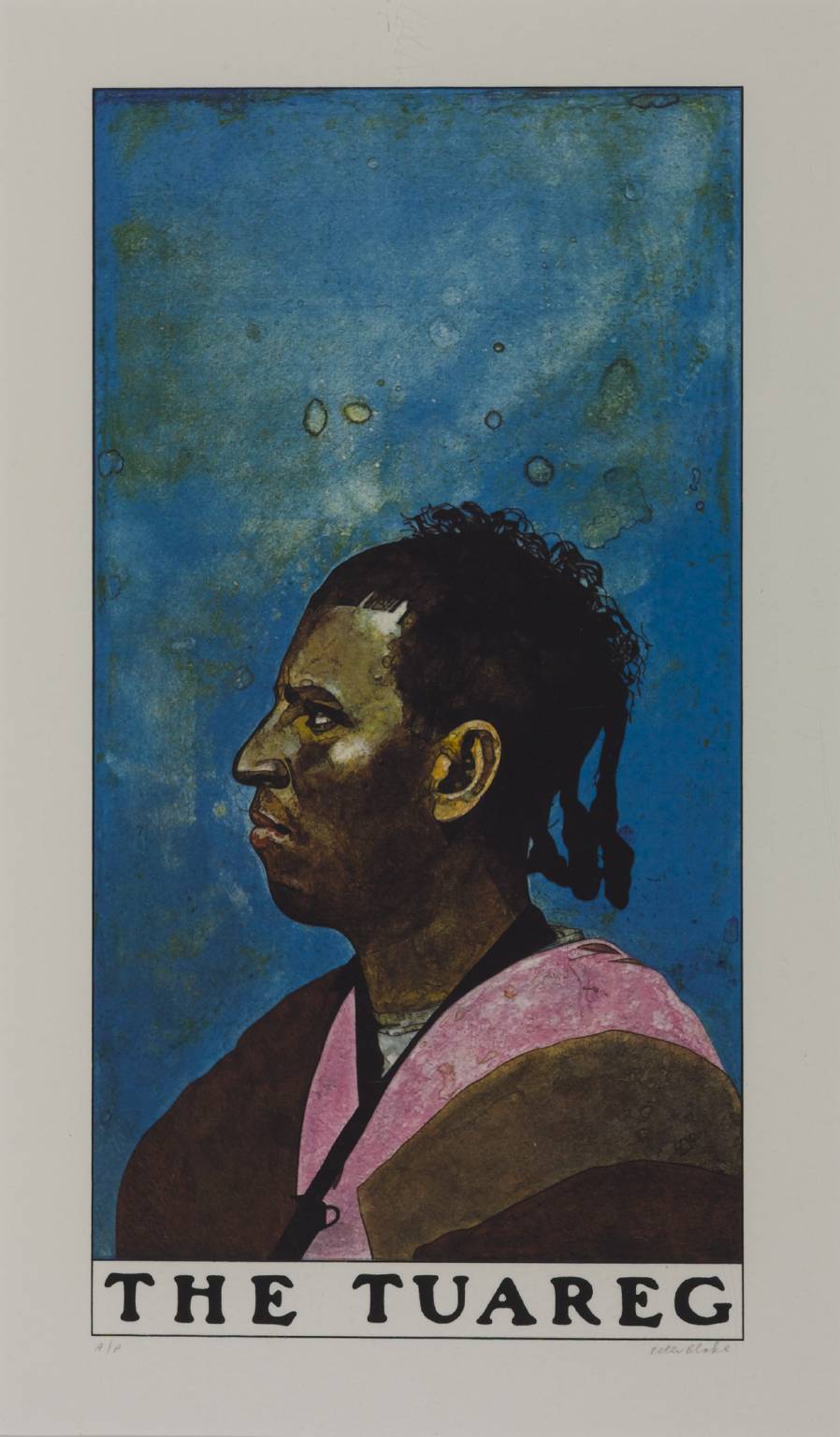The image depicts a detailed painting of an African-American man seen from the shoulders up, set against a medium blue background with muted green splotches that complement the overall composition. He has a stoic and serious expression, exuding a sense of nobility and regality. His hair is intricately styled with bangs combed down, curls on top, and braids hanging down the back. He is attired in a cape that drapes over his shoulders, characterized by light and dark brown shades with a dark pink stripe that crisscrosses in front. A black strap is visible around his neck. The man is positioned centrally in the image, looking off to the left side. At the bottom of the painting, the text "The Tatuareg" is inscribed, suggesting a possible tribal or cultural reference. The artist's signature is present but illegible.